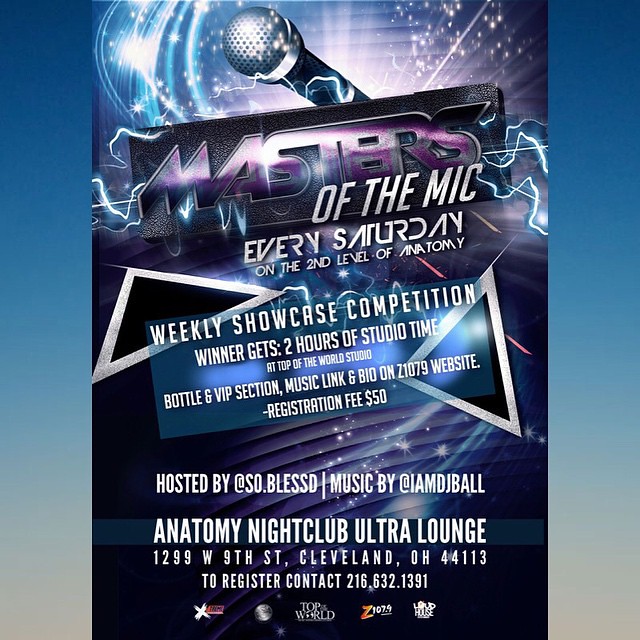The poster for a nightclub show features a vibrant blue background with dazzling white swirls, pinkish stripes, and sparkles at the very top. Dominating the black header with a purply chrome effect are the words "Masters of the Mic," accompanied by a prominent microphone design. Beneath this, it details that the event occurs every Saturday on the second level of Anatomy Nightclub. The middle section announces a "Weekly Showcase Competition," highlighting that the winner will receive two hours of studio time at Top of the World Studio, a VIP bottle service, and a music link and bio on the Z107.9 website. A registration fee of $50 is mentioned. The visuals include floating silver triangles, blue squares, and additional glitter stripes. Hosted by @so.blessd and with music by @iamdjball, the event is situated at Anatomy Nightclub Ultra Lounge, 1299 West 9th Street, Cleveland, Ohio, 44113. For registration, participants are instructed to contact 216-632-1391. Sponsors' logos, including Top World and Z107.9, are displayed at the bottom. The overall design exudes a futuristic aesthetic with striking blues, blacks, whites, and purples.